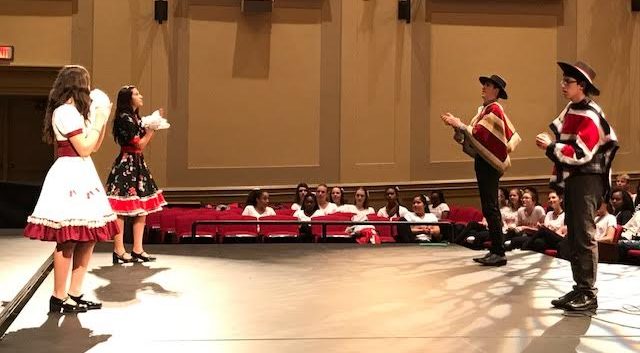This photograph features a vibrant dance performance captured on a white stage. At the center are two females and two males, separated into pairs with the women on the left and the men on the right. The females, dressed in multicolored Spanish dresses and black tap shoes, raise their hands as if clapping to the rhythm. The males don red and black ponchos, dark brown pants, and brown sombreros, also clapping along. Behind the performers, a diverse audience is seated in red chairs, watching intently from the ground level. The backdrop includes a brown wall, providing contrast to the lively scene on stage. The overall atmosphere emphasizes a traditional cultural dance performance, with an engaged crowd enhancing the authenticity of the moment.